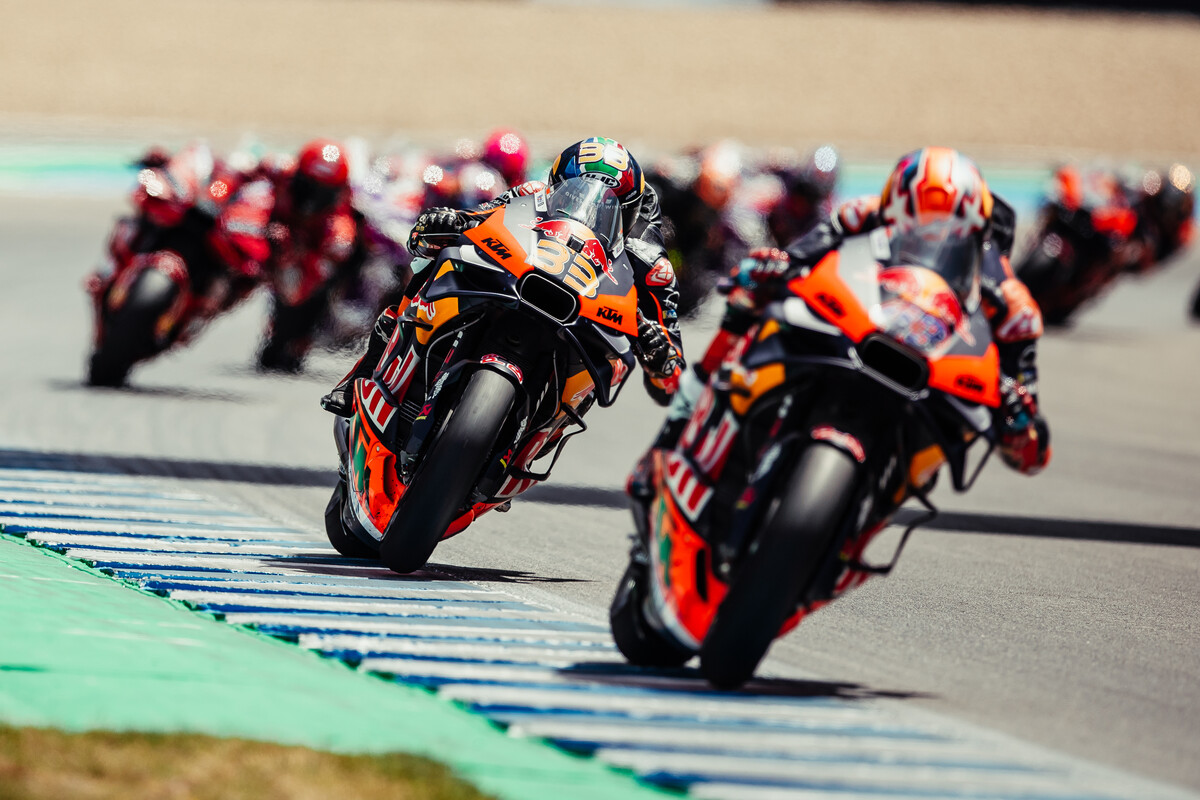The photograph captures a vibrant and dynamic moment from an outdoor motorcycle race on a bright and sunny day. The foreground prominently features two motorcyclists, skillfully maneuvering their black and orange motorcycles around a curve on the track. These two racers, who appear to be at the forefront of the competition, are incredibly detailed, standing out against a blurred backdrop of over ten other riders who fade into the distance.

The motorcycle leading the tight race on the right is ridden by a competitor wearing an orange and black helmet adorned with silver stars. This rider's gear consists of an orange-shouldered jacket, black sleeves, and matching orange gloves. In contrast, the racer on the left, closely contesting the lead, sports a helmet with a striking multi-colored design of blue, green, and red and carries the number 33. This second rider's attire features primarily black with two orange patches on the shoulders and black gloves. Notably, both motorcycles carry distinctive Red Bull logos prominently on their fronts. 

The track itself is well-defined, displaying a green-trimmed boundary with blue and white striped edges flanking the traditional gray asphalt. The action is centered as the riders tilt at an angle, navigating the turn with precision against a backdrop of greenery and blue pavement, capturing the intensity and excitement of the race.